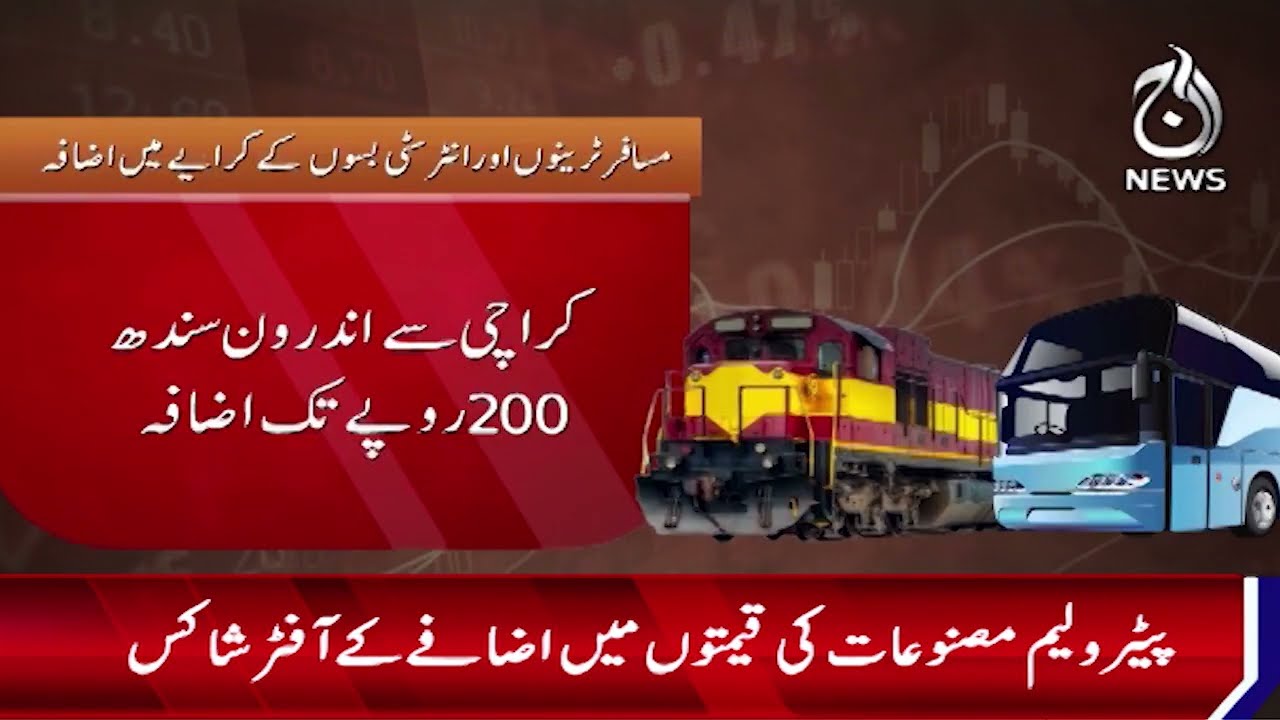The image appears to be a collage that serves as an advertisement or a news excerpt, prominently featuring elements related to transportation. It has a brown or black background and is filled with Arabic text. This text is spread across various sections of the image, including an orange background with white Arabic text in the left middle, and two lines of Arabic text on a red background along with the number "200" prominently displayed. At the bottom, there is another red background strip with white Arabic text.

In the upper right corner, there's a "News" label accompanied by a distinctive logo that resembles a curved teardrop or a dragon's tail. The visual elements include a colorful red and yellow striped train engine with a black bottom situated next to a blue and black bus. This imagery, combined with the use of Arabic script, suggests that the graphic could be an advertisement for transportation services, possibly for bus and train tickets, or a news segment focusing on travel updates. Overall, the image is rich in detail with a significant emphasis on Middle Eastern text and symbolic logos.